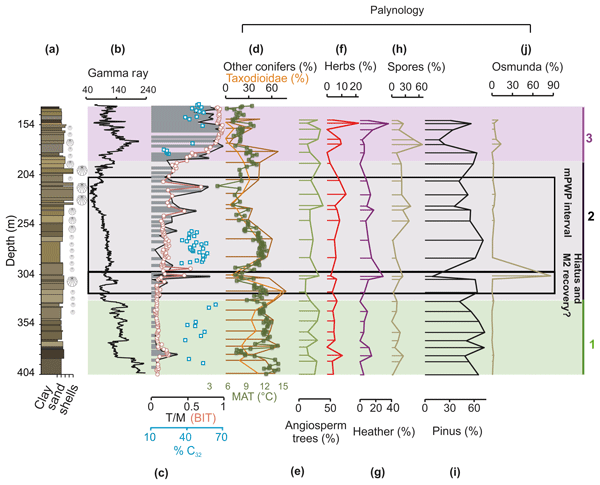The image is a detailed scientific chart titled "Palynology" at the top, illustrating data related to trees and plants. It features a main vertical line, branching horizontally, marked on the left with letter labels: A, B, D, F, H, and J. Under the label B, it lists "gamma ray," while D is followed by categories including other conifers, herbs (percentage), spores (percentage), and osmunda (percentage). The chart is segmented into three sections, each marked with numerical ranges from 154 to 404, and measures elements such as clay, sand, and shells on the far left with zigzagging lines in various colors (black, green, red, purple) indicating data trends. The far right side notes "hiatus" and "M2 recovery". Detailed numerical values like 41, 40, 240, and percentages (e.g., 0, 30, 60, 90) are provided under the gamma ray and other categories, with brown and purple areas providing visual representation. The chart is encased in an oblong square with lines measuring size and time at the bottom.